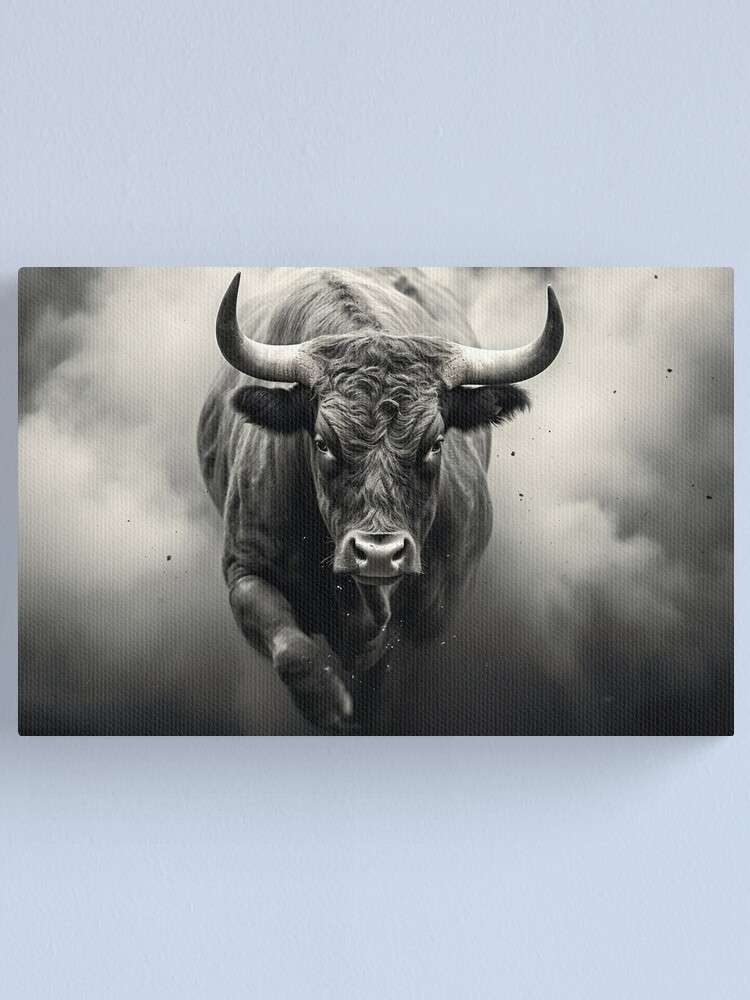The image is a detailed black-and-white drawing or AI creation of a black Angus bull charging directly at the viewer. Mounted in the center of a vertically oriented rectangle with a lavender-blue background, the bull stands out vividly. The bull's symmetrical horns are short and curved outward from either side of its forehead, slightly forward. Its eyes appear angry, and its thick, swirly forelocks and nose hair add to its fierce demeanor. The nostrils and nose are symmetrical, reinforcing the symmetry of the entire face. The bull's black ears jut out below the horns, complementing its powerful black body behind. One of its front legs is lifted, suggesting motion, with dust clouds and shadows swirling around it, enhancing the sense of speed and dynamism. The background features puffy, white dust clouds against a dark backdrop, giving the image a smoky, almost ethereal effect.